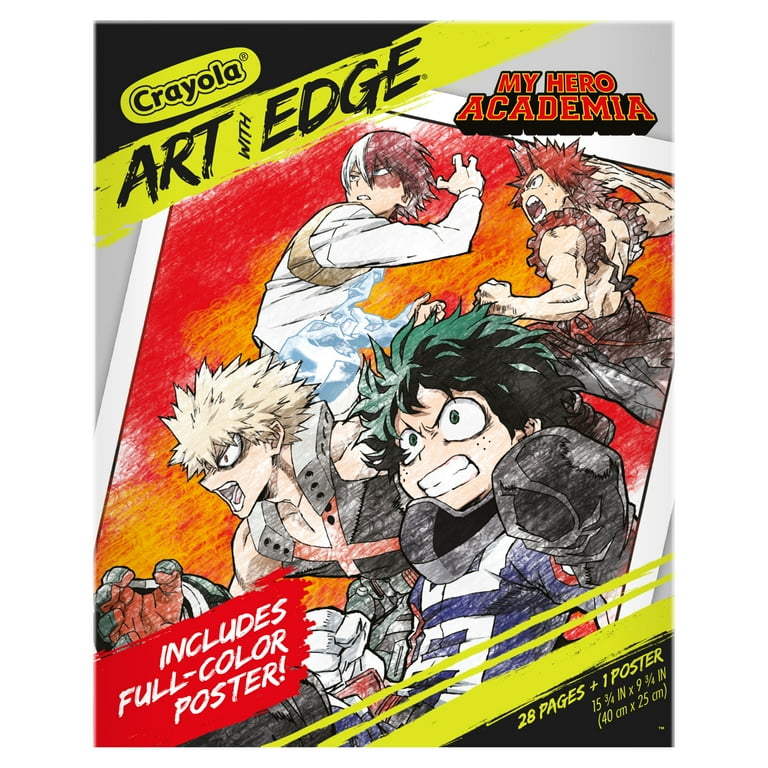This is a color-illustrated cover of a coloring book featuring characters from the anime series "My Hero Academia." The top left corner bears the text "Crayola Art with Edge," while to the right, the title "My Hero Academia" is prominently displayed. The cover showcases four vividly colored characters rendered with crayons or coloring pencils, all depicted in dynamic fighting stances with expressions of intensity and determination. The character at the top left has two-toned red and white hair and a distinctive port-wine birthmark under his left eye, striking a pose with his right hand raised. To his right, a young man appears mid-leap, his right arm pulled back as if ready to strike, with his left hand clenched. At the bottom left, a character with spiky blonde hair is shown facing downwards, his mouth wide open in a fierce yell. On the right, another young man with short green hair displays a resolute expression. The bottom left of the cover also highlights, "Includes Full Color Poster," and the bottom right specifies, "28 pages plus one poster, 15 3/4 inches by 9 3/4 inches, 40 centimeters by 25 centimeters." The overall design employs a stark and bold color scheme dominated by shades of yellow, red, and black.